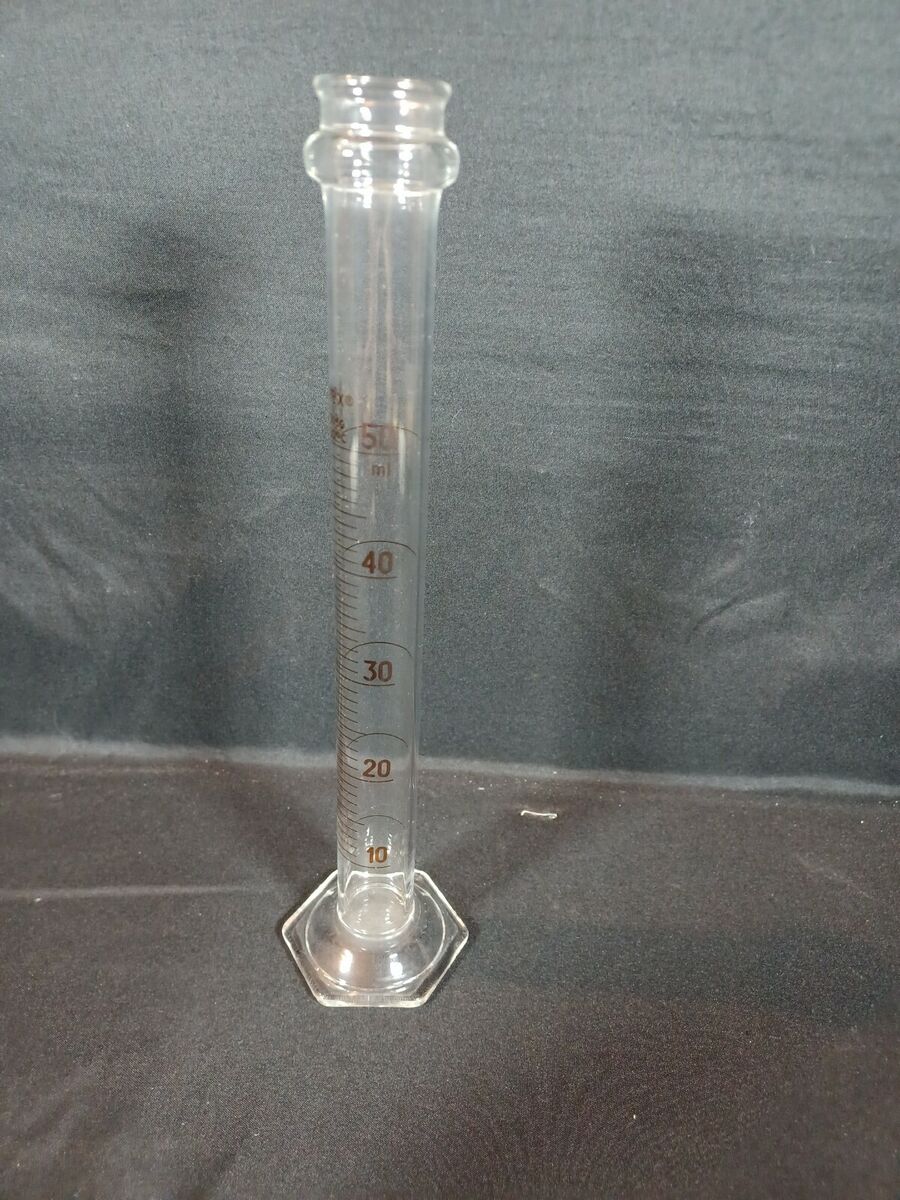The image captures a detailed scene featuring a tall, thin graduated cylinder, typically used in scientific experiments for measuring liquid volumes. The cylinder is clear and marked with measurement lines in milliliters, ranging from 10 at the bottom to 50 at the top, with increment markings at 10, 20, 30, and 40 milliliters. The top of the cylinder has a slight outward bevel. The setting appears carefully staged; the cylinder stands on a surface draped with a gray cloth, which extends into the background, imitating a painted backdrop but displaying evident wrinkles. Three shadows of the cylinder are noticeable: one to the left, one to the right, and another cast on the cloth-covered surface. The cylinder appears empty, and there is illegible writing near the measurement lines.